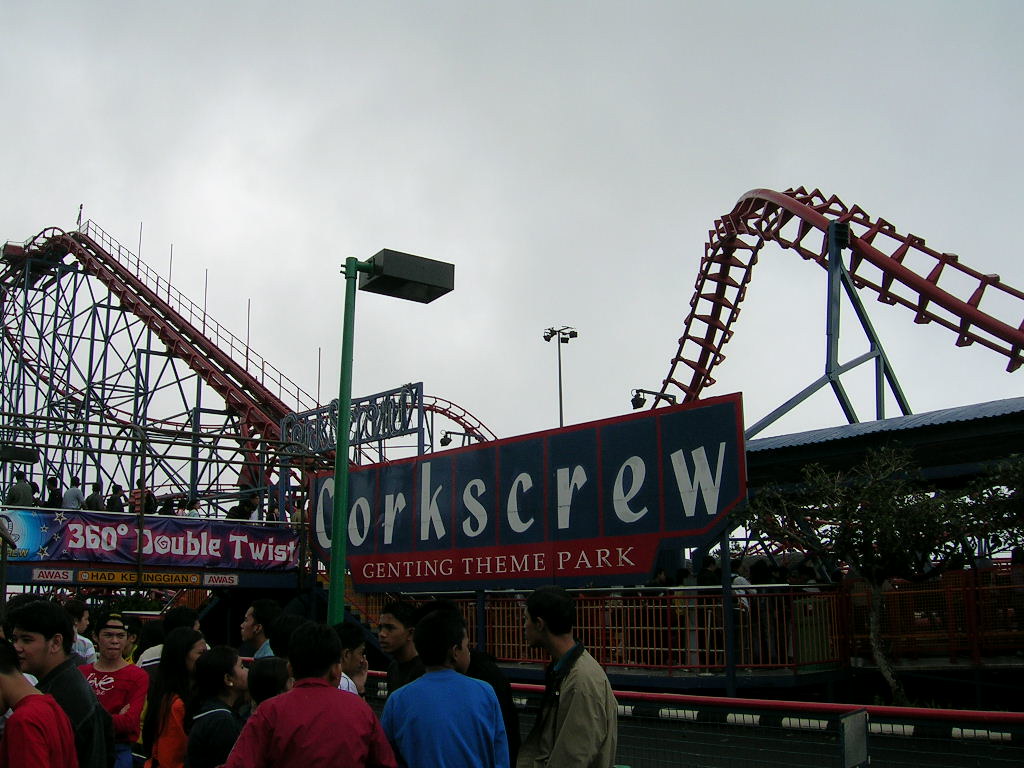This color photograph, taken in landscape orientation, captures a vibrant scene at Corkscrew Genting Theme Park. Dominating the foreground is a wooden banner, adorned with bold colors: "Corkscrew" in white against a blue background, and "Genting Theme Park" in white letters on red. The overcast gray sky adds a subtle contrast to the bright hues of the sign. To the side of the entrance, parts of the red-framed roller coaster, known for its thrilling 360-degree double twist, are visible in the distance. A green metal pole with a light fixture stands prominently at the front of the image.

A group of people, mainly young men and a few women, are seen milling about in front of the entrance, seemingly disorganized yet enjoying their time. Among them, identifiable figures include a young man in a blue long-sleeved shirt, another in a red long-sleeved shirt and a baseball hat, one in a green shirt, and another in a tan jacket. The backdrop includes two street lights, adding to the typical theme park ambiance. In the distance, the winding queue line for the roller coaster adds to the anticipation and excitement of this bustling amusement park scene.